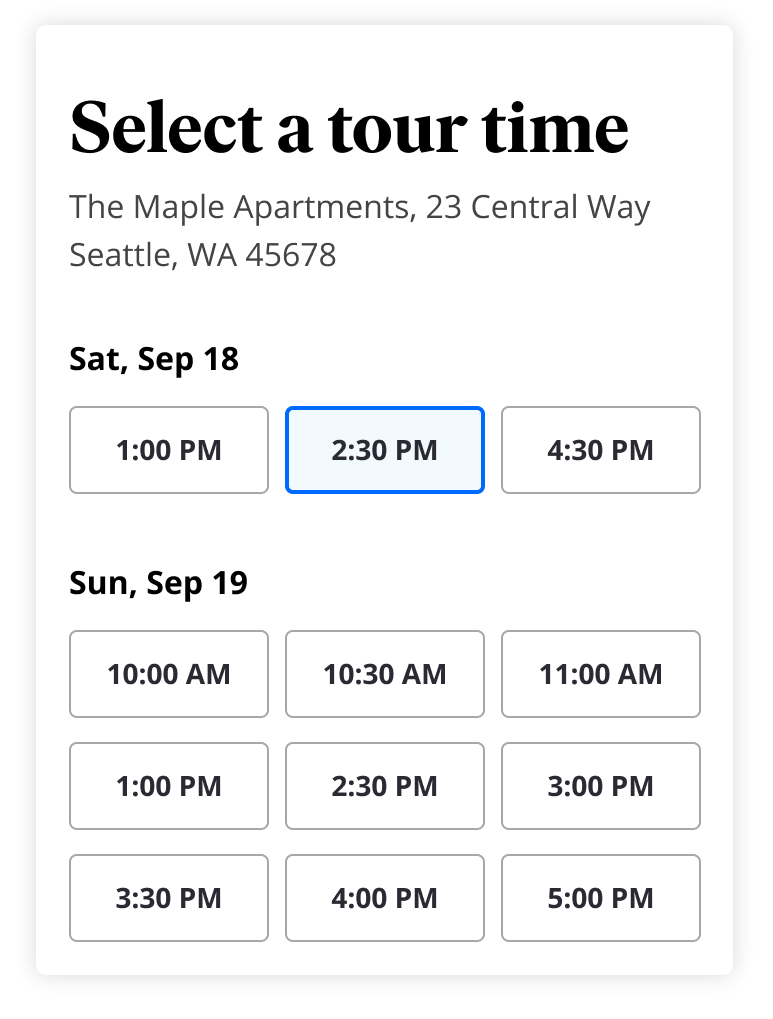The image displays a clean, white background with black text at the top that reads, "Select a Tour Time." Beneath this heading, the address "The Maple Apartment, 23 Central Way, Seattle, WA 45678" is prominently featured. Following the address, the text indicates "Saturday, September 18" with three available time slots. Each time slot is enclosed within horizontal black-outlined rectangles. The available time slots are 1 p.m. to 2 p.m., 2 p.m. to 3 p.m., and 4 p.m. to 5 p.m. The 2 p.m. to 3 p.m. slot is highlighted in blue, making it stand out from the others.

Below Saturday's schedule, "Sunday, September 19" is listed with six time slots: 10 a.m. to 11 a.m., 1 p.m. to 2 p.m., 2 p.m. to 3 p.m., 3 p.m. to 4 p.m., 4 p.m. to 5 p.m., and 5 p.m. to 6 p.m. These time slots are similarly enclosed in black-outlined rectangles but none are highlighted. In total, there are nine time slots presented across the two days with clear delineation and organization, enhancing readability and user convenience.